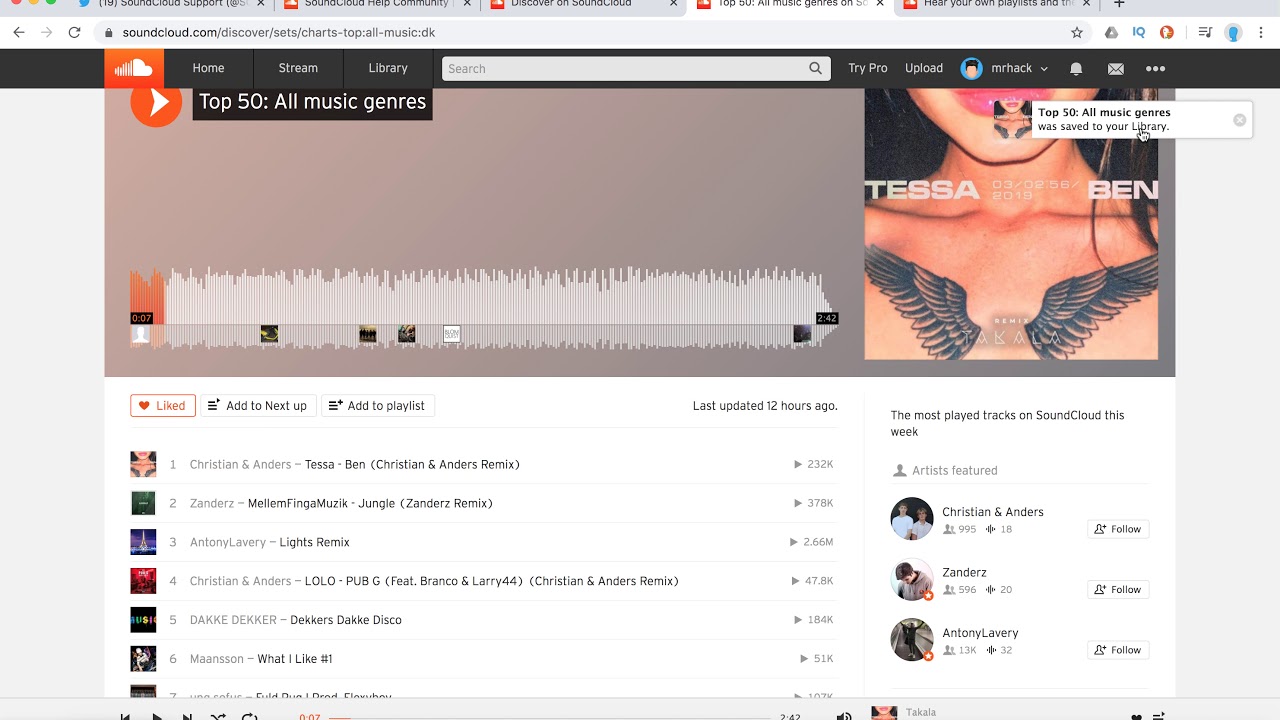This image is a detailed screenshot of someone's web browser, focused primarily on a SoundCloud page. In the top left corner, three circles—red, yellow, and green—indicate the window controls. To the right of these controls, five open tabs are visible. The first tab displays the Twitter logo, while the remaining four tabs exhibit the SoundCloud logo, suggesting that they are SoundCloud pages. The current active tab is the fourth one.

Below the tabs, the URL address bar shows the web address as soundcloud.com. To the left of the URL, standard navigational buttons are present: back, forward, and refresh. On the far right side of the URL bar, several browser extensions are visible, including Google Drive, iCue, and DuckDuckGo extensions.

In the main content area of the browser window, the SoundCloud website is displayed with a header titled "Top 50 All Music Genres." To the right of this title, there is a square image of a woman labeled "Tessa Ben." The lower section of the image showcases several smaller square thumbnails, each representing different artists and their songs. The first thumbnail features "Tessa Ben," followed by "Jungle," "Lights Remix," "Local PUBG," and "Deckers Drake Disco."